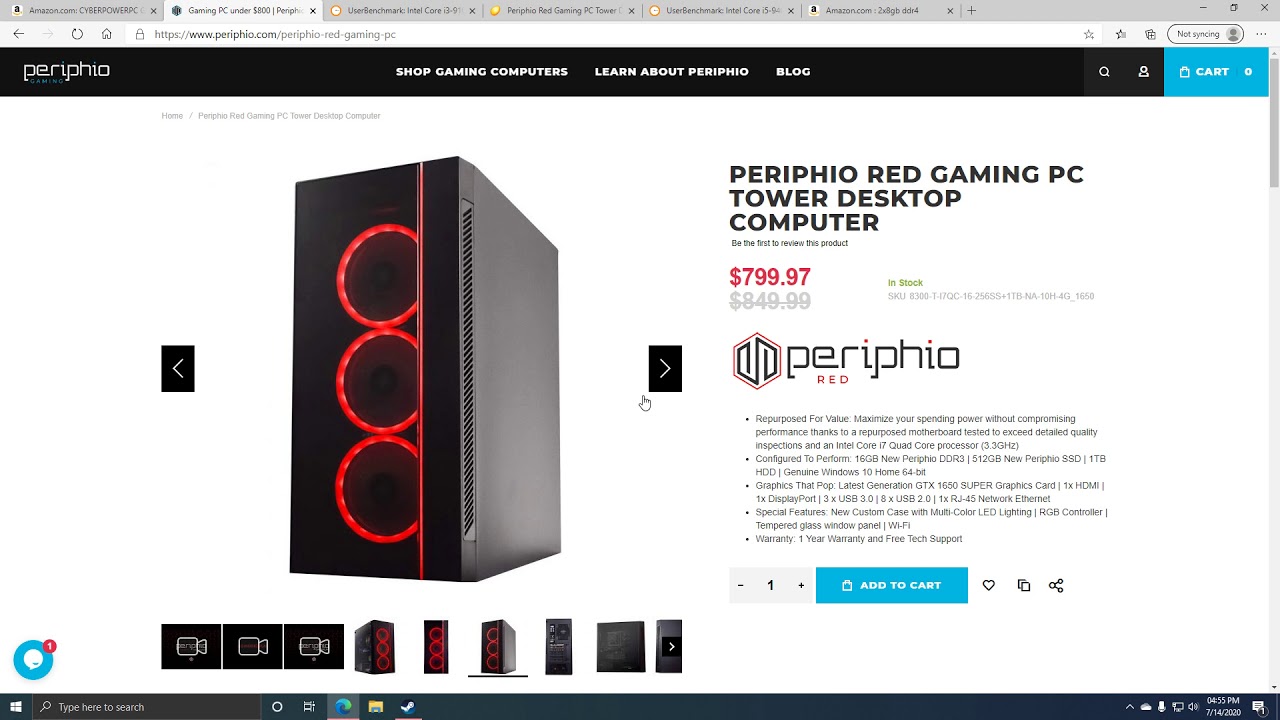The image depicts a screenshot of a web browser displaying the Perifio website. At the top of the screen, there are six tabs open, although their titles are too small to read clearly. The URL bar shows "https://www.peripi.com" twice.

The Perifio website features a sleek black navigation bar at the top. Positioned centrally on this bar are the options: "Shop Gaming Computers" in white, "Learn About Perifio," and "Blog" in white.

The central section of the page highlights a prominent image of a black gaming PC tower, equipped with three fans illuminated by red LED lights. This setup is advertised as the "Perifio Red Gaming PC Tower Desktop Computer." To the right of the image, the price is indicated as a range from $799.97 to $849.99, signifying it is on sale and currently in stock. Below the main image, there is a brief, though difficult to read, description of the product.

Directly beneath the featured image, there is a carousel of additional images available for scrolling. The screenshot also shows the Windows taskbar at the bottom of the screen, typical of a PC interface.